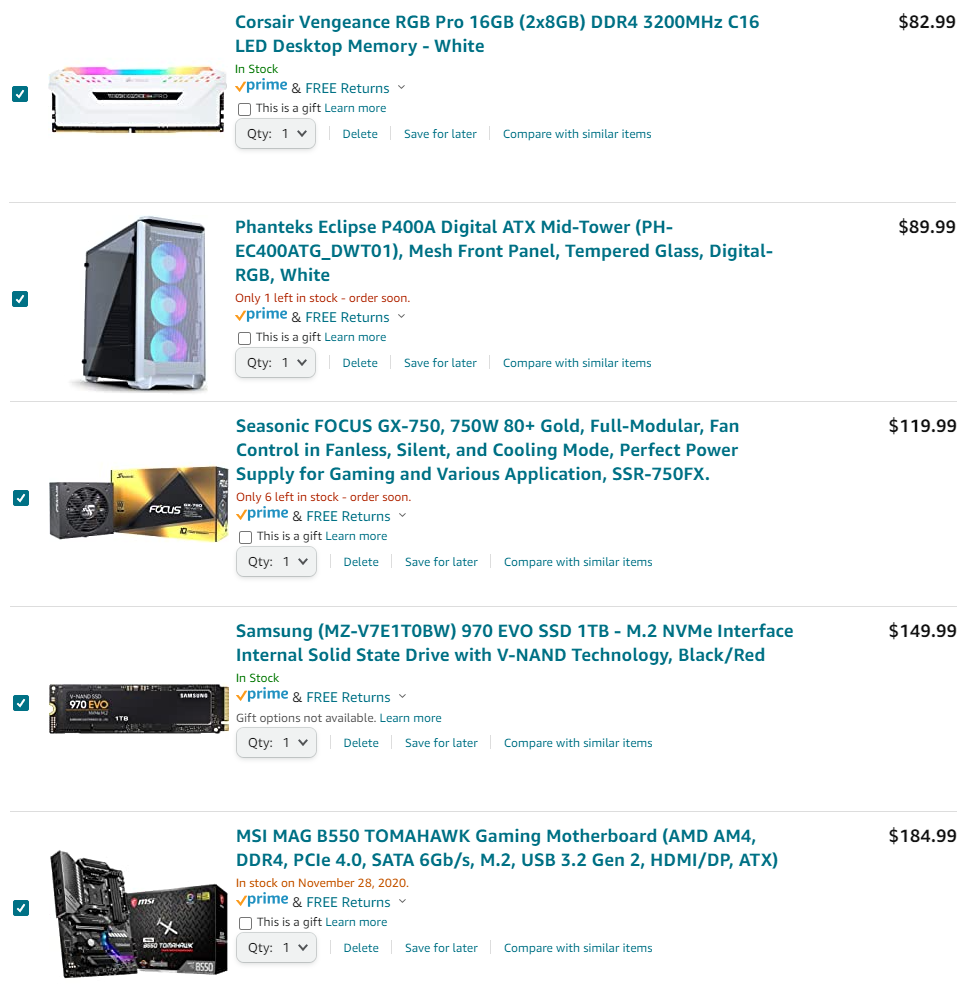A detailed and descriptive caption for the image would be:

---
The image showcases a high-quality Corsair Vengeance RGB Pro desktop memory stick. This RAM module, which is pre-installed, features a striking white design with vibrant RGB lighting at the top, making it a standout component for any build. Specifically, it's a 16GB kit consisting of 2x8GB sticks, supporting DDR4 at 3200MHz with C16 latency. This product, labeled 'Dash White,' is known for its performance and aesthetics, priced at $82.99.

Additionally, there's a sleek Phanteks Eclipse P400A digital ATX mid-tower PC case, also in white, designed for efficient airflow with a mesh front panel and tempered glass side. The case features integrated digital RGB lighting, making it a perfect match for the illuminated RAM. 

The setup is powered by a Seasonic Focus GX-750 power supply. This 750W unit, priced at $119.99, offers 80 Plus Gold efficiency, full modularity, fan control modes, and operates silently, making it ideal for gaming and other demanding applications.

For storage, a Samsung 970 EVO 1TB NVMe M.2 internal solid-state drive is included. Utilizing V-NAND technology, this SSD offers high-speed data transfer rates, providing ample storage at $149.99.

Lastly, the components are installed on an MSI MAG B550 Tomahawk Gaming Motherboard. This motherboard supports AMD AM4 processors, features PCIe 4.0, SATA 6Gb/s, dual M.2 slots, and multiple USB 3.2 Gen 2 ports, ensuring robust performance and connectivity for gaming and other intensive tasks.

Together, these components create a powerful, visually stunning, and highly functional PC build.